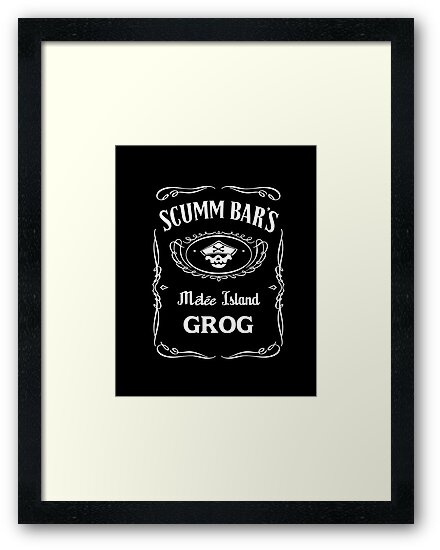The image is a wall hanging or picture frame with a black border. Inside, there is a large white space surrounding a central black rectangular box. This box features predominantly white text and designs. At the top of the rectangle, in a curved font, it says "Scum's Bar." Below that, "Melee Island Grog" is written in smaller white text. In the center is an oval emblem containing the skeletal head of a pirate wearing a hat adorned with a crossbones symbol. This emblem is surrounded by intricate, ornate white designs that give the image a pirate-themed aesthetic, reminiscent of a redesigned Jack Daniels label. The picture is likely a custom-made piece for someone's home bar, evoking a sense of adventure and maritime lore.